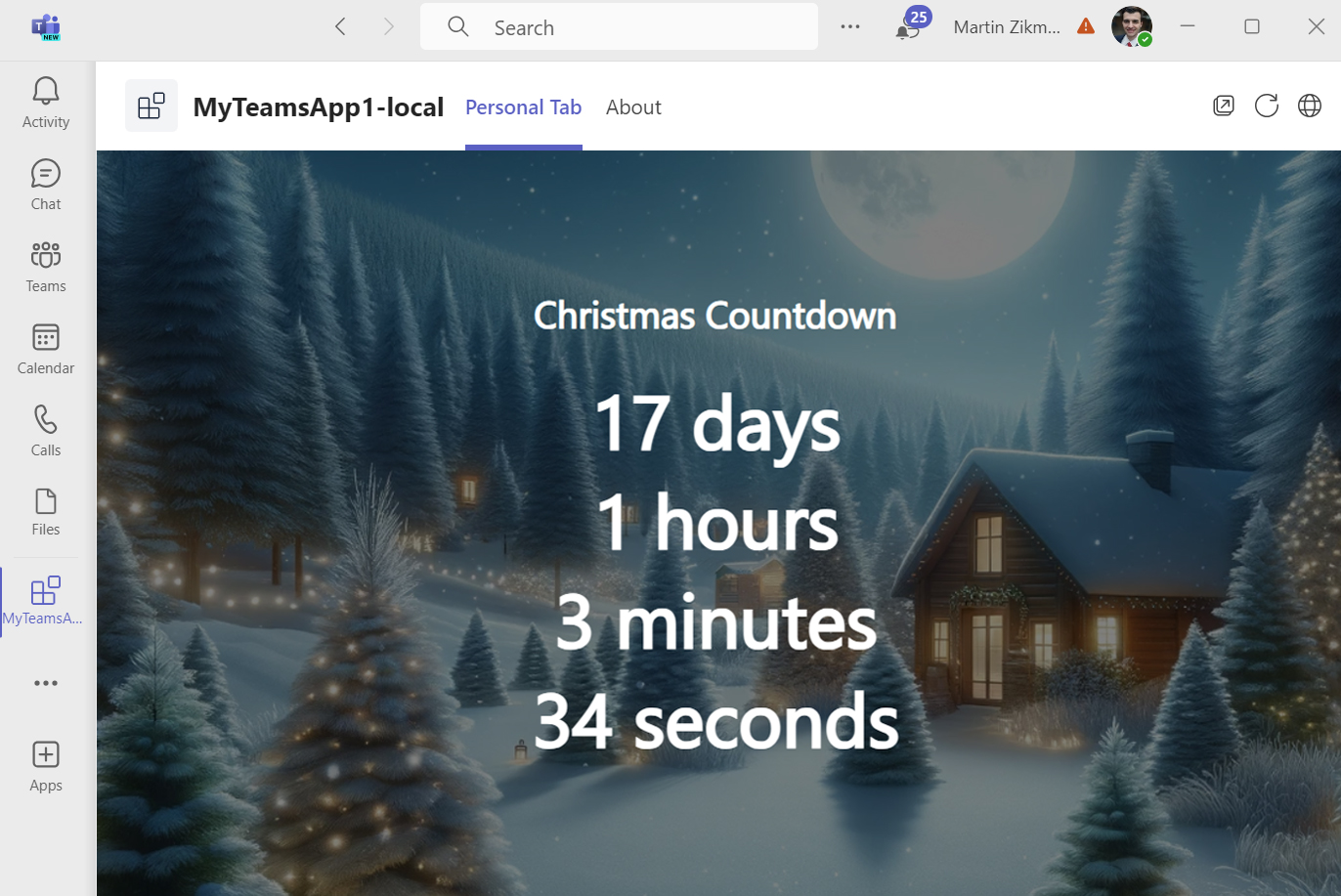The image depicts a website screen featuring a detailed user interface layout. On the left side of the screen, a vertical menu displays categories in the following order: Activity, Chat, Teams, Calendar, Calls, Files, with 'My Team A' selected, followed by the Apps section. 

At the top right of the screen, a set of elements includes a search bar, a notification icon showing 25 notifications, the profile user name, and controls for minimizing, maximizing, and closing the window.

Directly underneath, the header text reads "My Teams App, 1-Local" in black, accompanied by two tabs: a blue-highlighted 'Personal' tab and a black 'About' tab. Three small icons are positioned to the right of these tabs, with a refresh icon centered among them.

Beneath this header is a section displaying a Christmas countdown timer set to 17 days, 1 hour, 3 minutes, and 34 seconds. 

The background image is an animated winter scene featuring a brown house with a snowy roof and illuminated windows emitting a warm yellow glow. The house, seen from the front and right side, is surrounded by snow-covered trees adorned with lights. Above the serene landscape, a vast blue sky is dominated by a large, white moon.